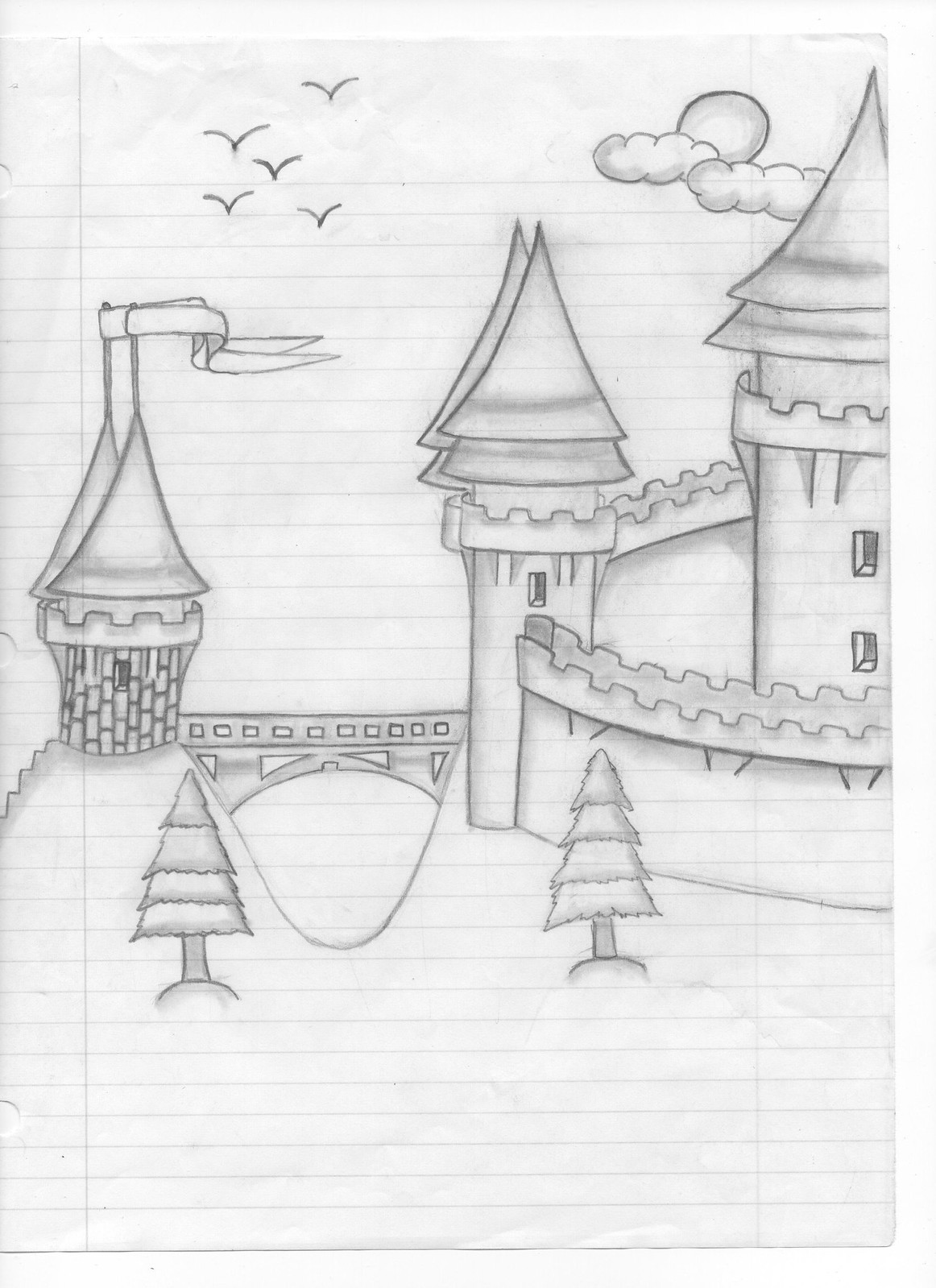The image is a detailed pencil sketch on a piece of standard notepad paper, characterized by its vertical margin line on the left and horizontal lines intended for writing. In the drawing, a castle stands prominently in the middle of the page. The castle has three main towers – one on the left, one in the center, and one on the right – each paired with a second, slightly hidden tower behind them. The towers on the left feature two slender, horizontal flags waving in the wind. 

The sky in the upper left-hand corner of the sketch contains five bird-like V shapes arranged like the sides of a die, while the upper right-hand corner depicts a circular shape, which could be interpreted as either the sun or the moon, accompanied by two clouds. Below this celestial detail, the castle is flanked by a visible bridge on the middle left and two small hills with trees at the base of the image. The entire scene, captured on the lined paper, brings a whimsical, storybook-like quality to the sketched castle landscape.